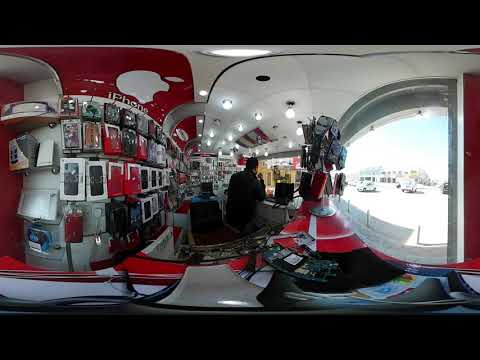The photograph depicts the interior of an Apple store, presumably in a foreign country given the unrecognizable script beneath the iconic white Apple logo on the red wall. The store's decor prominently features an interplay of red and white, with circular white bulbs dotting the ceiling. The left-hand side showcases a wall adorned with dozens of vertically rectangular packages, likely containing various Apple merchandise such as phone cases and other accessories. In the center, there is a man dressed in dark clothing, standing behind a counter cluttered with electronics, potentially including keyboards and tablets. To the right, large windows flood the store with daylight, revealing a parking lot outside where several cars are parked near a two-story building. The image is captured with a fisheye lens, distorting proportions and giving a comprehensive 360-degree view of the indoor-outdoor environment of the small mall area where this retail store is situated.